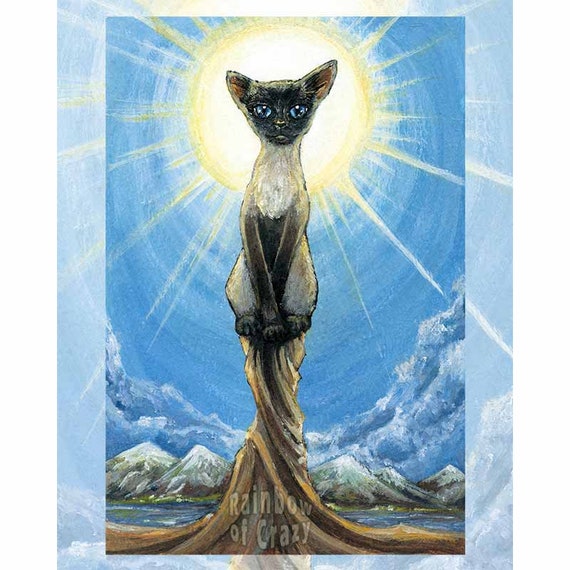This is a detailed, poster-sized painting of a Siamese cat with blue eyes, perched on a tall, twisted wooden base that resembles tree roots. The cat has a sleek black body and a white fur neck. It is set against a vibrant blue sky dominated by a large, radiant golden sun with rays extending in all directions. Below the cat and sun, there are white, snow-capped mountains and clouds arranged in a semicircular pattern. The entire scene is enclosed within a light blue border, with additional clouds depicted at the bottom edges. At the bottom of the painting, there is a curved watermark that reads "Rainbow of Crazy."